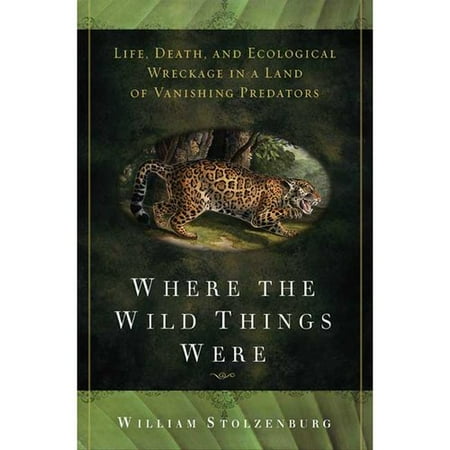The cover of the book features a vibrant and intricate design. The top and bottom borders showcase a textured pattern resembling a large, green leaf, adorned with elegant ink designs. Dominating the central portion is a splotchy black and dark brown mosaic with an oval inset at its heart. This oval contains an exquisite illustration of a leopard, poised to pounce, with a large tree looming behind it. Above the oval, in light green text, is the phrase "Life, Death, and Ecological Wreckage in the Land of Vanishing Predators." Beneath the illustration, in bold white font, reads the title "Where the Wild Things Were." At the bottom of the cover, the author's name, William Stolzenberg, is elegantly printed in white.